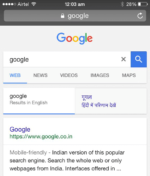In this screenshot from a mobile device, the status bar at the top indicates a strong network signal with 4 to 5 bars, suggesting a stable connection. The screenshot was taken at 12:03 AM, as shown in the center of the status bar. The device appears to be an iPhone, with the battery level at approximately 20%, and the Bluetooth icon visible at the top right.

The main screen displayed is a Google search page. Prominently featured is the Google logo, along with a search field where text has been inputted. Below the search field, various categories are listed, including News, Videos, Images, and Maps. Only one search result is visible in the screenshot, a link to Google, indicated as being from google.com with a ".co.ir" domain extension. The screenshot effectively captures a moment of browsing within the Google search interface on an iPhone late at night.